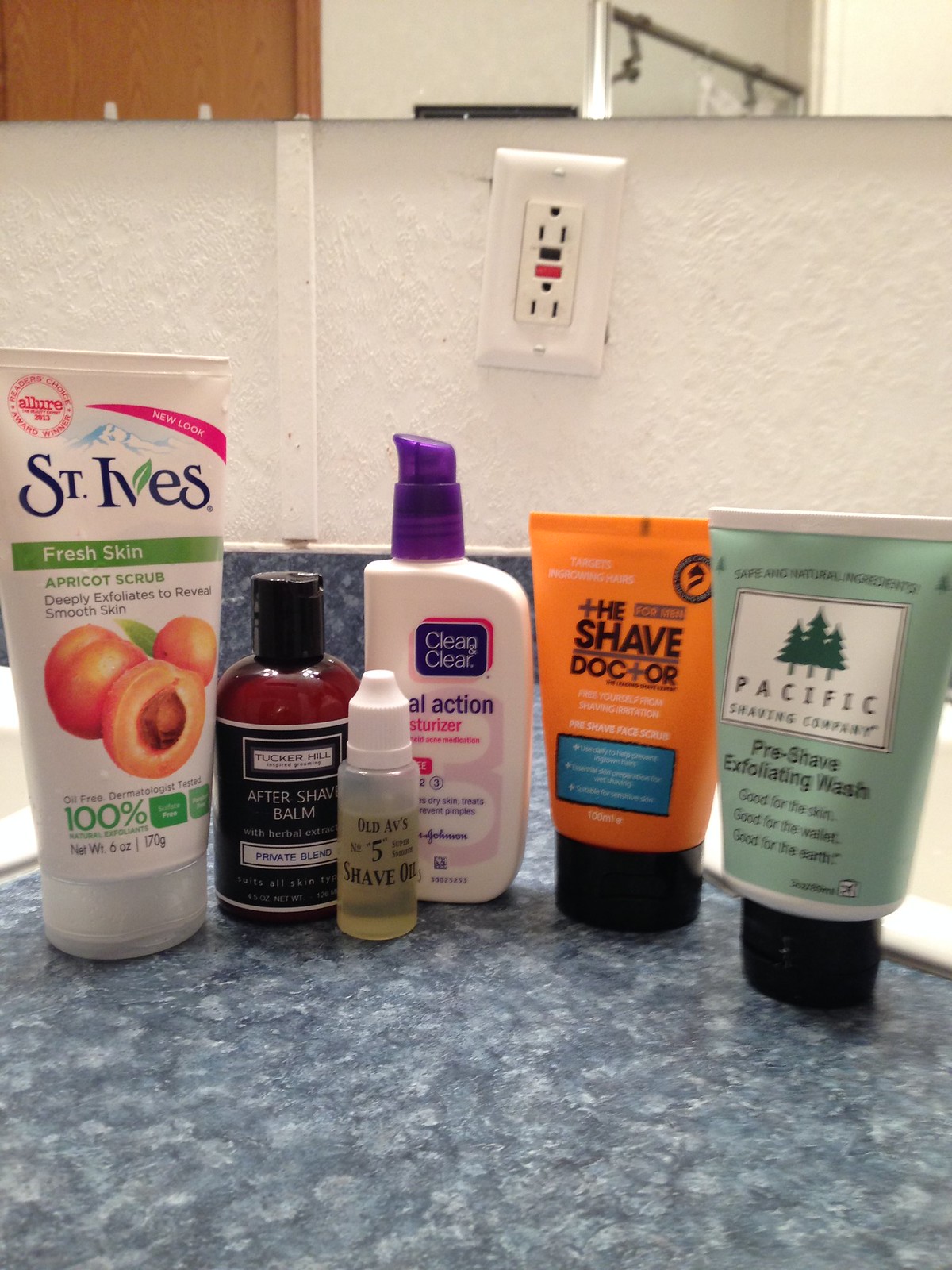A detailed arrangement of skincare products adorns a blue marble-patterned countertop. The countertop gracefully curves up to meet a white, slightly stucco-textured wall. A white strip runs vertically, leading up to a power outlet featuring two slots. Above this outlet, a glimpse of a brown door, a white room, and an open doorway reveals a metal banister sloping downward.

The countertop hosts six distinctive skincare products lined up from left to right. First, a St. Ives Fresh Skin Apricot Scrub in a white tube with a matching cap. An illustration of apricots, one of which is halved to reveal its pit, decorates the tube. Next, a bottle of aftershave balm stands with a black label, white text, and red liquid sealed by a black cap. Following that is a tiny, slim bottle with a white cap, containing yellow liquid, likely shaving cream. Beside it, there's a moisturizer topped with a striking purple cap. Finally, two tubes complete the lineup: one orange with a black cap labeled "The Shave Doctor," and another sage green with black cap, featuring tree illustrations, labeled as pre-shave exfoliating wash.